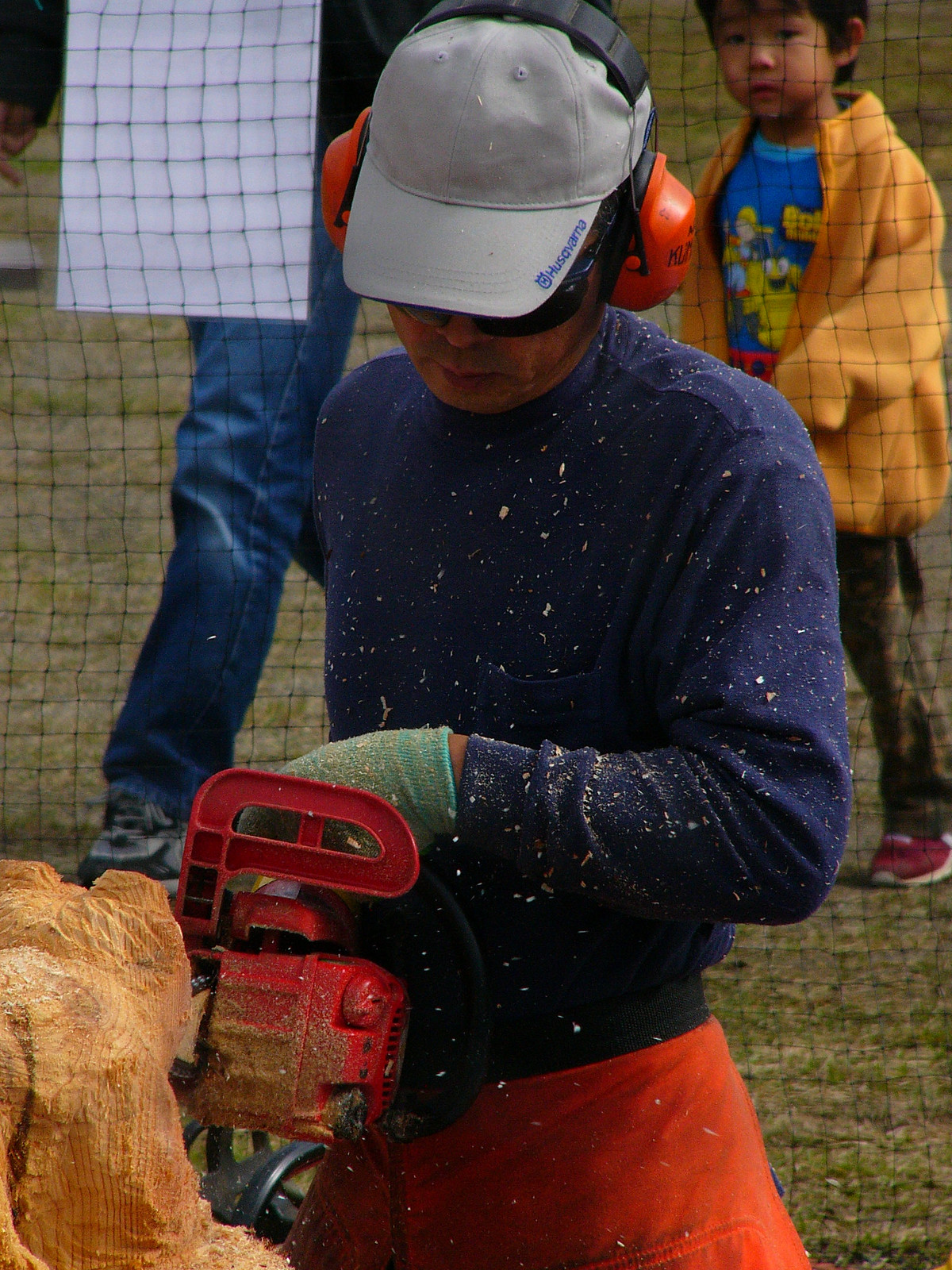The photograph captures a logger actively carving a curved wooden sculpture using a red chainsaw. The man, dressed in protective gear, including orange earmuffs, black sunglasses, a gray baseball cap with blue text spelling "Husqvarna," a long dark blue shirt, and burnt orange pants, stands behind black netting. His attire is further accessorized with blue gloves, and greenish sawdust speckles his clothing. The light brown and orange-hued wood artifact is partially visible in the foreground, evoking an artistic design. A curious young boy, dressed in a yellow fleece and camouflage pants, along with an adult wearing blue jeans and a black shirt, stands near the fence in the background. Sawdust created by the chainsaw flies onto the logger’s clothes as he meticulously works on the sculpture.